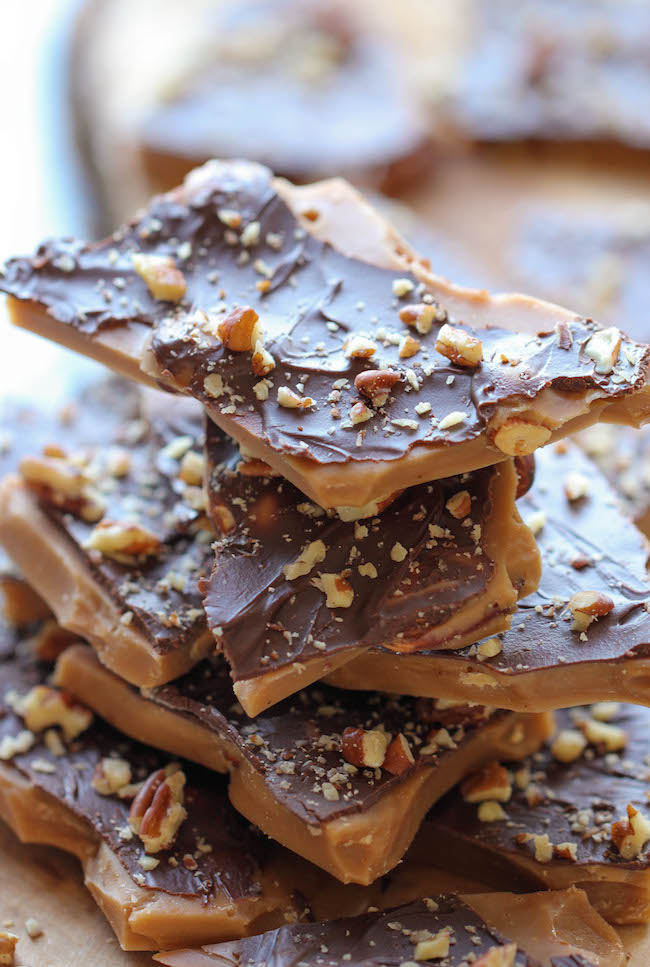The image features a detailed close-up of a stack of approximately ten freshly-baked, homemade caramel cookies. Each cookie has a light brown caramel base, is coated with a thin layer of dark chocolate, and is sprinkled with small pieces of nuts, likely a mix of pecans and almonds. The cookies are intricately cut into rectangular slabs and meticulously stacked on top of each other. The foreground brings the stack into sharp focus, while the background is blurred but suggests an abundance of additional cookies, reinforcing the scene's rich, decadent atmosphere. The cookies rest on a wooden surface, further adding to the homemade, rustic feel of the image, and they appear irresistibly fresh, ready to be enjoyed.